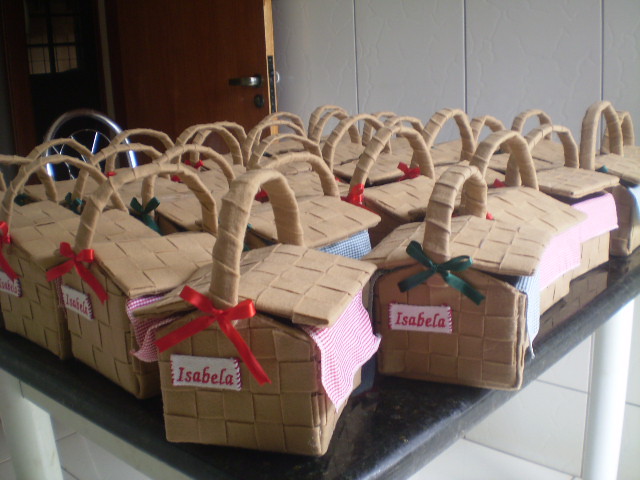The image depicts a daytime indoor setting with a table covered in numerous handmade, light brown baskets resembling gingerbread house shapes. Each basket, constructed from interwoven strips of wood, features a hinged opening on both sides, a handle tied with ribbons—green on the left and red on the right—and a checkered cloth (either white-and-red or blue-and-red) draped from it. All baskets are labeled with the name "Isabella," spelled I-S-A-B-E-L-A. The table is set against a backdrop of a white-paneled wall, a wooden door with a silver handle, and a chrome-colored chair. The scene is captured in a rectangular photograph.